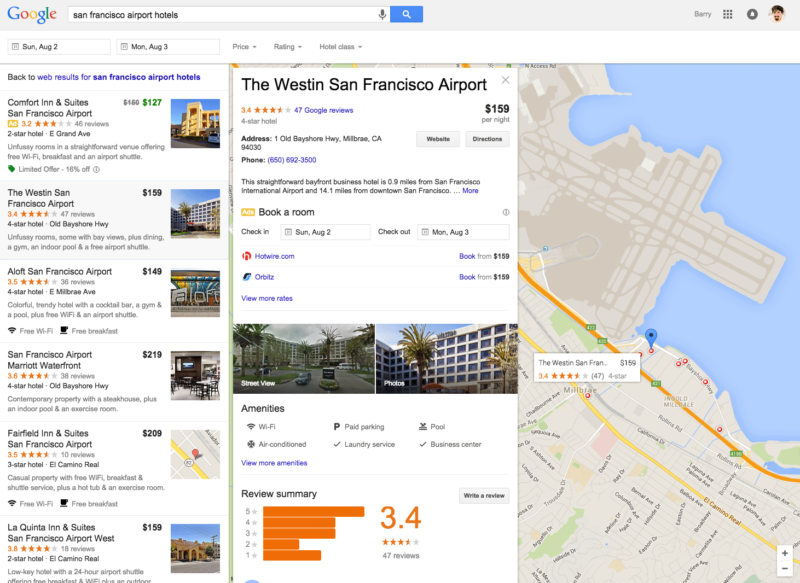The image depicts a Google search results page for "San Francisco Airport Hotels." The search query and the results are visible in a web browser, with the Google logo prominently displayed in its characteristic blue, red, yellow, and green colors in the upper left corner. The search bar shows the query, "San Francisco Airport Hotels," and the dates from Sunday, August 2nd to Monday, August 3rd.

The results display various hotel options with images, names, prices, ratings, and booking options. The highlighted hotel is The Westin San Francisco Airport, showing a larger image alongside its details. 

Other hotels listed include:
- Comfort Inn and Suites San Francisco Airport
- The Westin San Francisco Airport
- Aloft San Francisco Airport
- San Francisco Airport Marriott Waterfront
- Fairfield Inn and Suites San Francisco Airport (which displays a map instead of a hotel image)
- La Quinta Inn and Suites San Francisco Airport West

The Westin San Francisco Airport is highlighted with the following details: the price per night is $159, it has received 47 Google reviews, and holds a rating of 3.4 stars. Further information includes booking options via Hotwire and Orbitz and a link to "View More Rates." Amenities and a summary of reviews are listed, and additional images of the hotel are displayed.